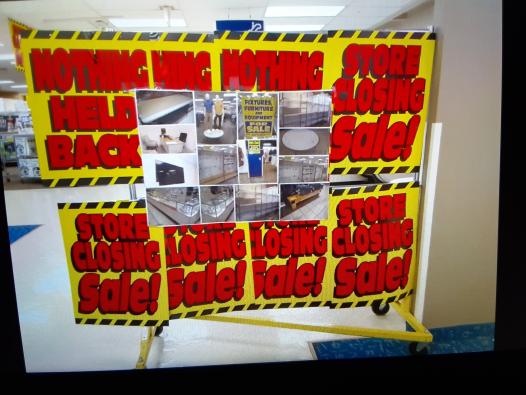The photograph captures an advertising sign on display in a store, set against a background of a white tile floor and a drop ceiling with fluorescent lights. The sign, mounted on a yellow rack with black wheels, features a prominent yellow hue accented with black and yellow caution stripes. Bold red text on the sign reads, "Nothing held back" and "Store closing sale." This message is repeated multiple times across eight poster-like signs, creating an urgent and compelling visual. The setting reveals additional details, such as a small section of blue carpet seen in the right-hand corner, and portions of blue squares on the floor. The scene includes shelves with items and square light fixtures on the ceiling, emphasizing the typical store environment. The sign's yellow frame and strategic placement near store counters and a doorway underscore the gravity of the store's closing sale. The central part of the sign showcases twelve images depicting various store interiors, including racks and tables, adding context to the sales event.